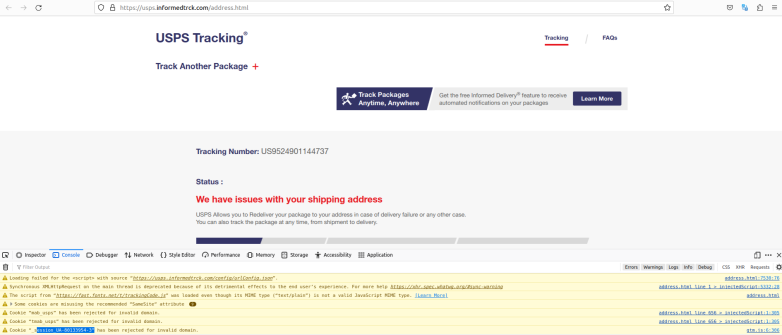This image depicts a screenshot of the United States Postal Service (USPS) website, specifically the USPS Tracking page. The page highlights several key features and functionalities, including the ability to track packages and the option to sign up for the "Informed Delivery" feature, which provides automated notifications regarding the status of your parcels. The tracking information shown includes a sample tracking number, US9524901144727, with a status update indicating issues with the shipping address. The USPS offers solutions for delivery failures, such as re-delivery to the intended address. Additionally, there are technical details visible in the console, reflecting loading scripts and issues with cookies, including one script loaded with an invalid JavaScript type and multiple cookies missing the recommended SameSite attribute, leading to rejections.